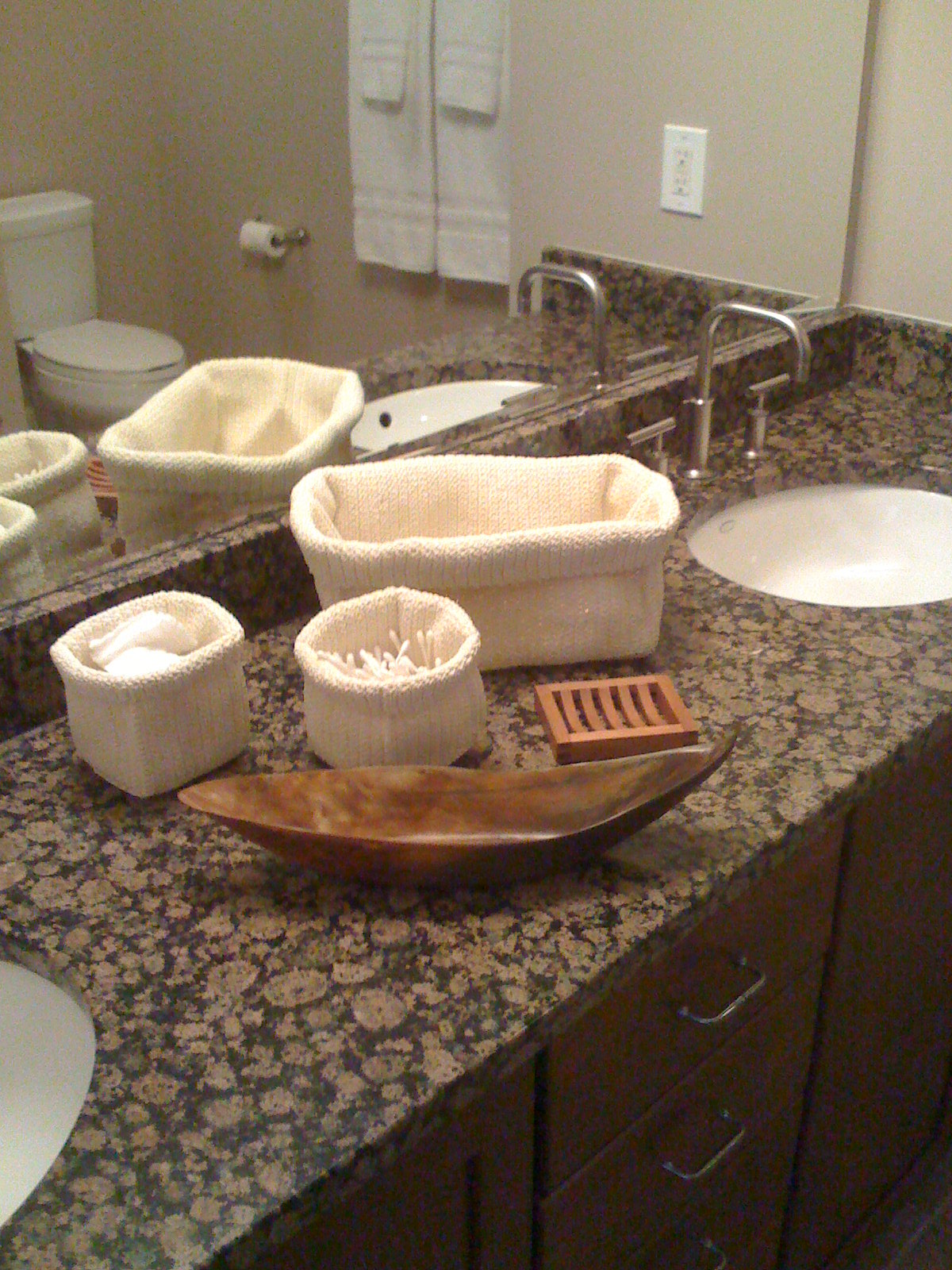The photograph captures a well-organized bathroom countertop featuring a rich, dark brown set of drawers and cabinets beneath. Centered drawers are accented with sleek silver pull-out handles, enhancing their modern appeal. The countertop itself is an elegant display of dark brown and light brown granite, characterized by a predominantly dark background interspersed with large tan splotches. 

Two sinks are positioned on either side of the countertop; the left sink is partially visible, while the right sink, complete with a silver metal faucet and handles, is more prominently displayed. Between the sinks, three light tan cotton fabric baskets are arranged. One rectangular basket is flanked by two more rounded square baskets, one filled with q-tips and the other with white cotton pads. Adding to the decor, a wooden banana leaf-shaped tray and a square wooden coaster are also centrally placed on the countertop.

In the reflection of the mirror, additional bathroom elements such as a toilet, a toilet paper roll, and hanging towels can be seen, adding depth and a sense of completion to the overall scene.